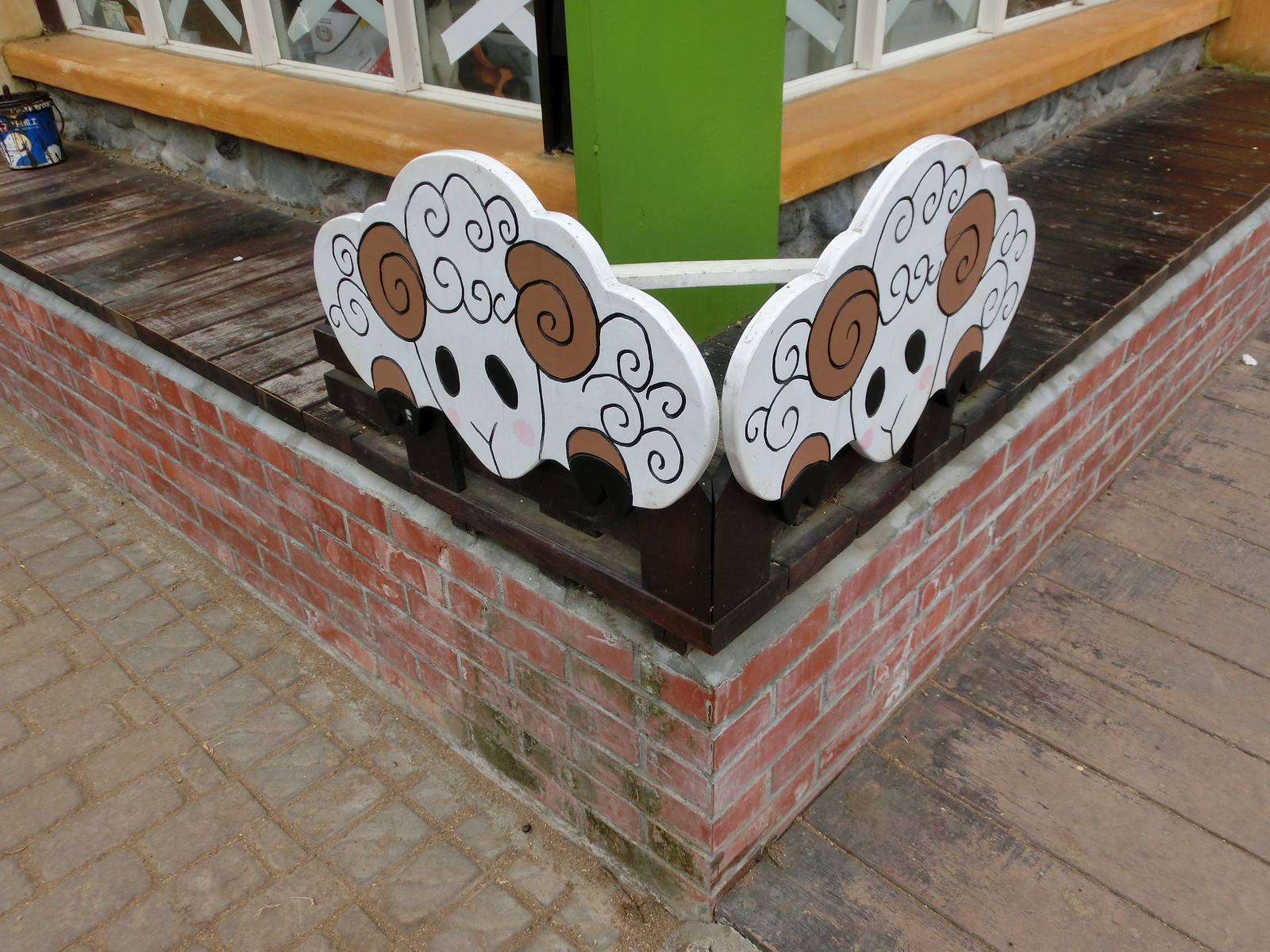The image depicts an outdoor scene taken from the perspective of someone standing at a corner where two different types of walkways meet. On the right-hand side of the image, there is a wooden walkway made of horizontal wood planks. On the left-hand side, there is a stone walkway with grayish stones separated by a brown sandy material. In the center of this corner, there is a very short red brick wall transitioning from wood on the right to stone on the left, forming a pointed shape where the walkways converge. Atop the brick wall is a layer of dark wood slats, possibly forming a small elevated structure.

Prominently featured in the corner and leaning against a green beam are two white wooden decorative sheep. Each sheep has black swirling lines depicting wool, brown swirls suggesting horns, black eyes, and a bit of pink on the cheeks. The sheep appear to be fastened together around the middle with a white bar, and they sit on wood paneling. One sheep faces the wooden walkway while the other faces the stone walkway. In the background, there appears to be a light-colored structure with windows.